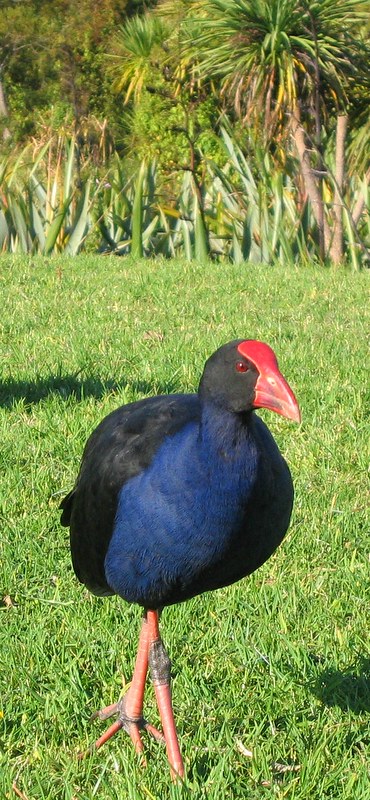In the vibrant image, a striking bird with a bright red eye showcases a captivating blend of colors. Its chest features a light blue reminiscent of a blue crayon, while its head is a contrasting black adorned with a vivid red beak. The bird's upper plumage transitions to darker shades of blue and black, complementing its orange-hued legs streaked with black markings. Sharp claws are visible at the ends of its toes as it meanders through a lush green field. The background is rich with natural elements, including a palm tree and various greenery, interspersed with shadows cast by unidentified structures or people, adding depth and context to the serene scene.